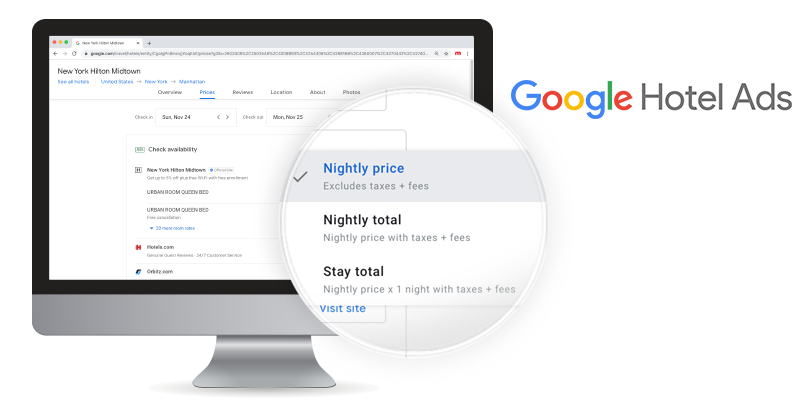This image is part of a Google Hotel ad campaign. The iconic "Google" logo features its characteristic colors: blue for "G," red for "O" and "E," yellow for the second "O," and green for "L." A large computer monitor is prominently displayed on the left side, showcasing various details about a hotel booking interface. Overlapping the monitor, a magnifying glass zooms in on a specific section of the screen for emphasis.

The background monitor replicates a typical computer interface, complete with three colored buttons—red, yellow, and green—located in the top left corner. The open window on the screen indicates a booking for the "New York Hilton Midtown." The interface displays several navigation tabs: "Overview," "Prices" (highlighted), "Reviews," "Location," "About," and "Photos." 

Key booking details are visible: check-in on Sunday, November 24th, and check-out on Monday, November 25th. There's an option to check availability, and the hotel’s offer includes an "Urban Room, Queen Bed" with free cancellation. Price listings from Hotels.com and Orbitz.com are also mentioned.

The magnified section highlights a confirmed selection with a check mark next to the "Nightly Price" (excluding taxes and fees). Additionally, there is information about the "Nightly Total," which includes the nightly price with taxes and fees and the total cost for one night's stay.

This detailed depiction aims to give potential customers a comprehensive view of the booking process and pricing transparency for the New York Hilton Midtown.